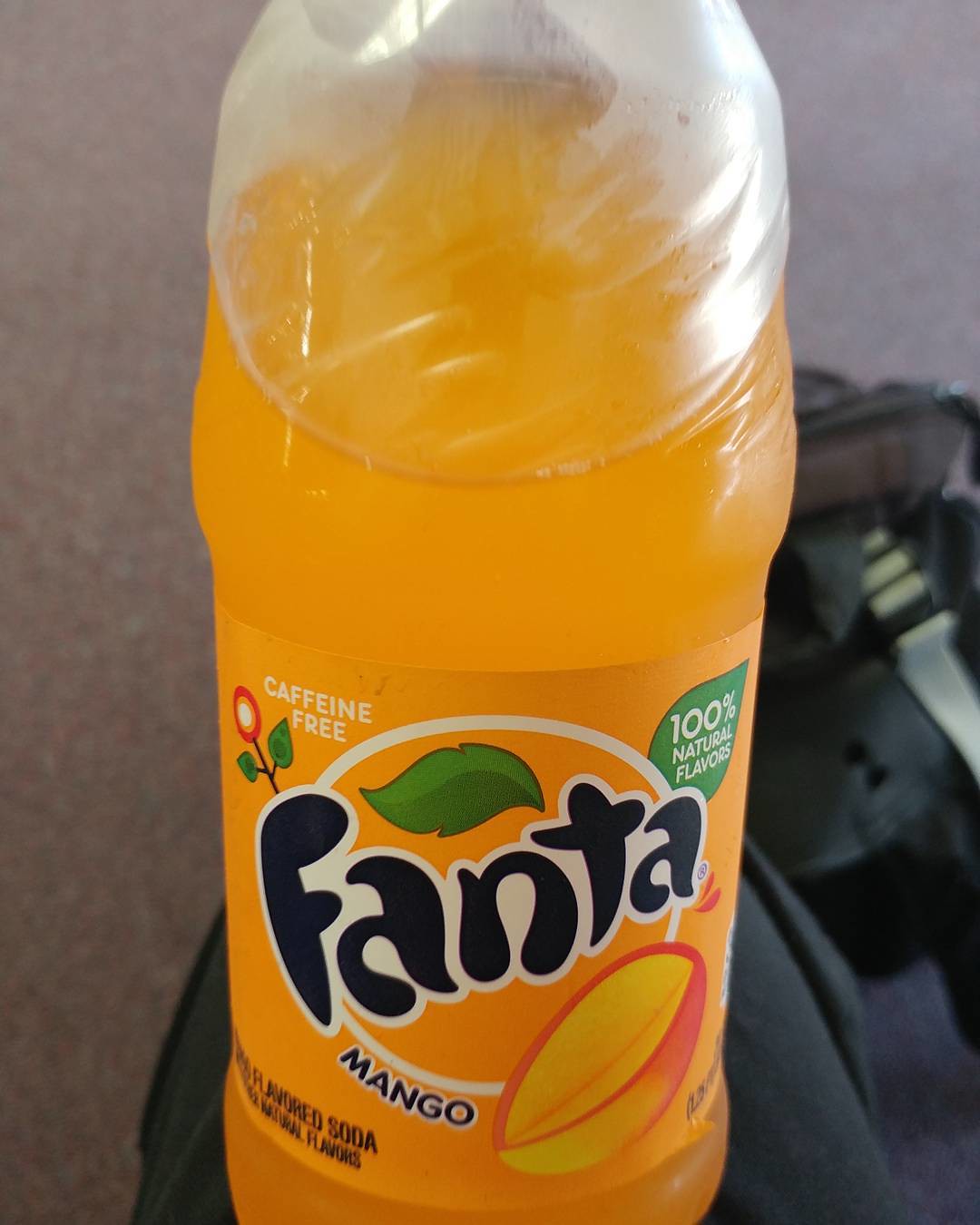This photograph features a clear bottle of Fanta Mango soda, distinguishable by its vibrant orange hue, which extends from the bottle's label to the drink inside. The prominent Fanta logo appears in bold white letters set against an orange backdrop, complemented by a white circle. Above the logo, a green leaf adds a fresh touch. Below, the word "Mango" and an image of a halved mango highlight the flavor. To the top right, a green leaf and the text "100% Natural Flavors" emphasize the drink's natural ingredients. On the top left, a circular red flower with two green leaves and the phrase "Caffeine Free" in white lettering indicate the beverage contains no caffeine. Additionally, the bottom left corner of the label displays the words "Flavored Soda" in black ink.